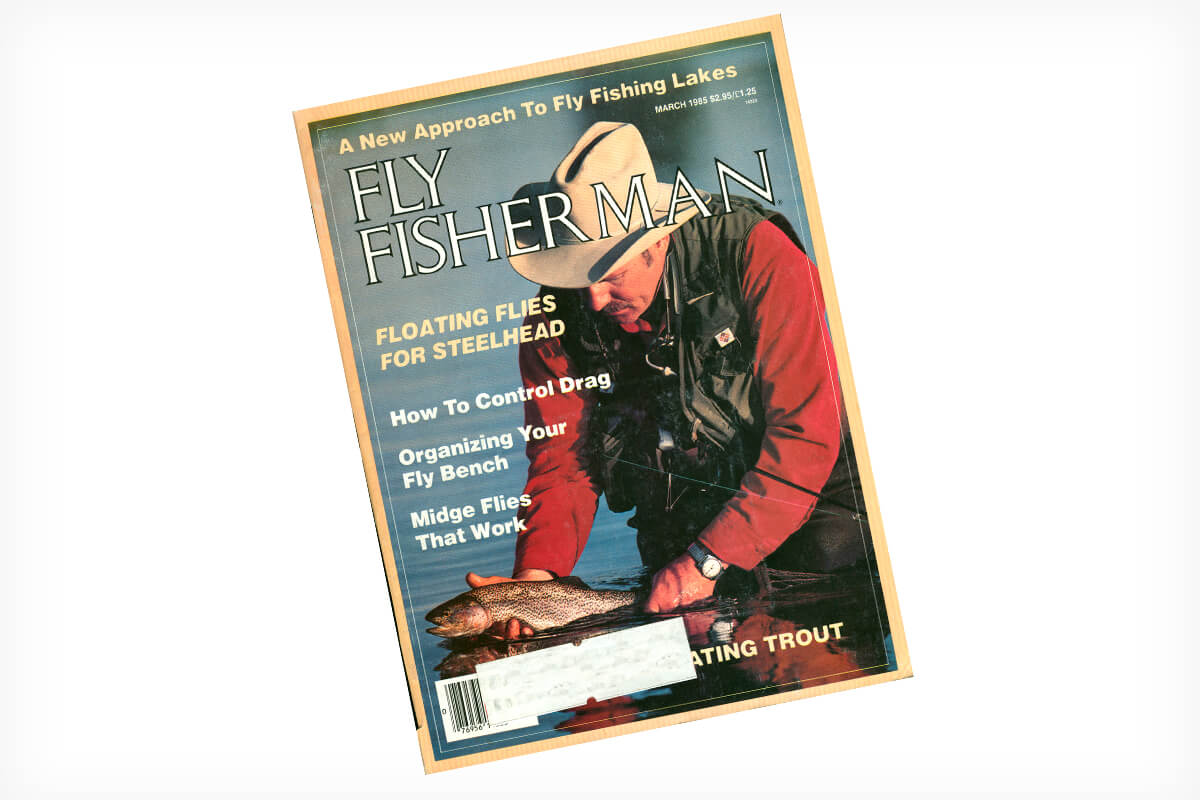The image is a tilted photograph of the "Fly Fisherman" magazine with the cover date partially obscured. The headline reads "A New Approach to Fly Fishing Lakes," suggesting a focus on lake fishing techniques. The cover features articles including "Floating Flies for Steelhead," "How to Control Drag," "Organizing Your Fly Bench," and "Midge Flies that Work." The bottom left hosts a UPC code, and a digitally blurred mailing label is visible near it. The cover photo shows a man, waist-deep in water, wearing fly fishing gear, including a beige cowboy hat, a long-sleeved dark red shirt, a black fishing vest, and a wrist watch on his left wrist. He cradles a speckled trout in both hands, poised to release it back into the water. The man’s attire and the fish together evoke the practical and immersive experience of fly fishing.